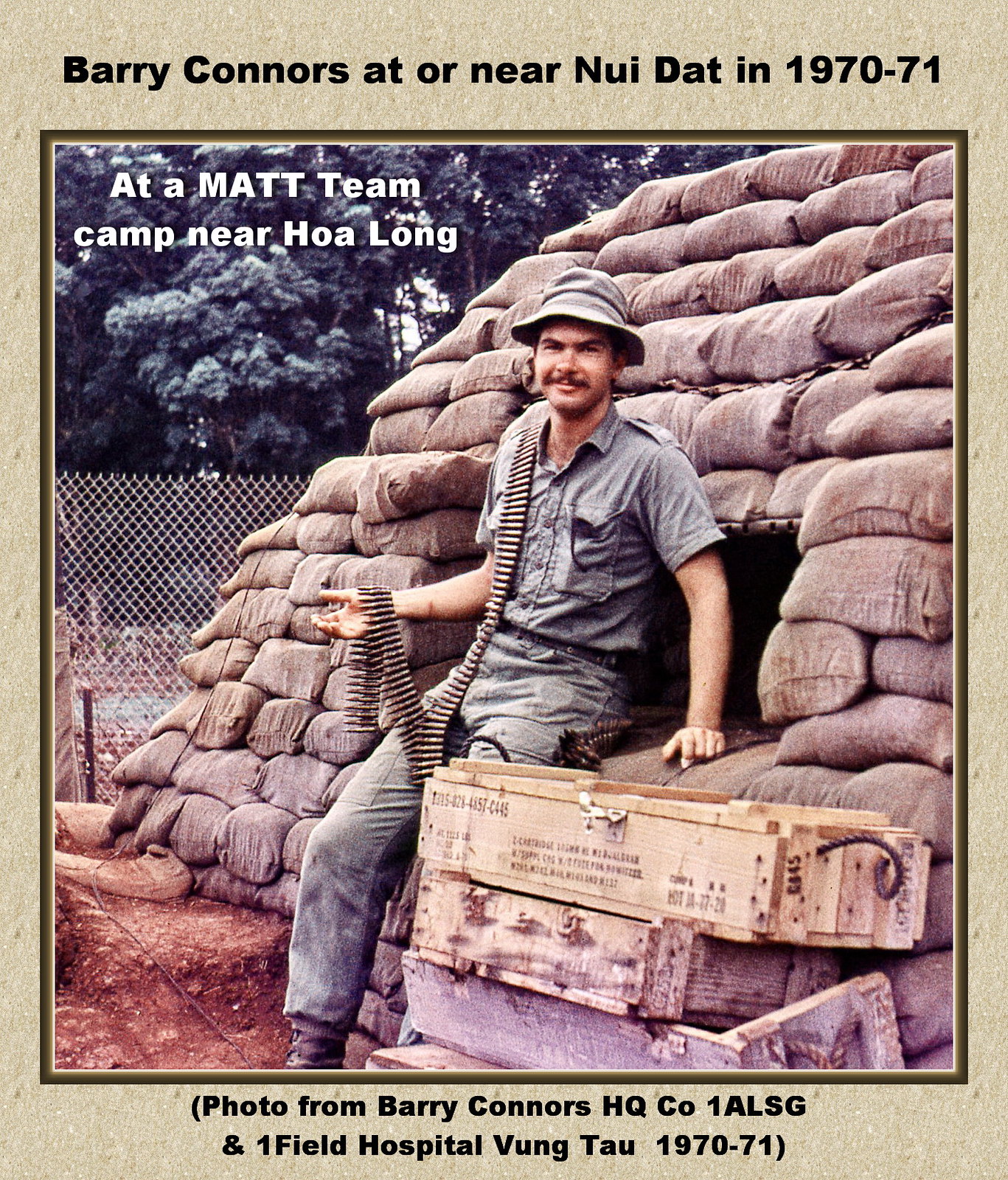This poster features a photograph of a soldier identified as Barry Connors, taken at or near Nui Dat during 1970-71. In the image, Barry is seated against a wall of sandbags that form a makeshift shelter. He is dressed in a hat, short-sleeved shirt, and long pants, with ammunition draped over his right shoulder and held in his hand. To his left, there are wooden crates stacked together. The background includes a large tree and a fence. Above the picture, text reads "Barry Connors at or near Nui Dat in 1970-71," and in the upper left-hand corner, it says, "At a MAT team camp near Hoa Long." The bottom of the poster notes, "Photo from Barry Connors HQ CO 1 ALSG and 1 Field Hospital Vung Tau 1970-71."